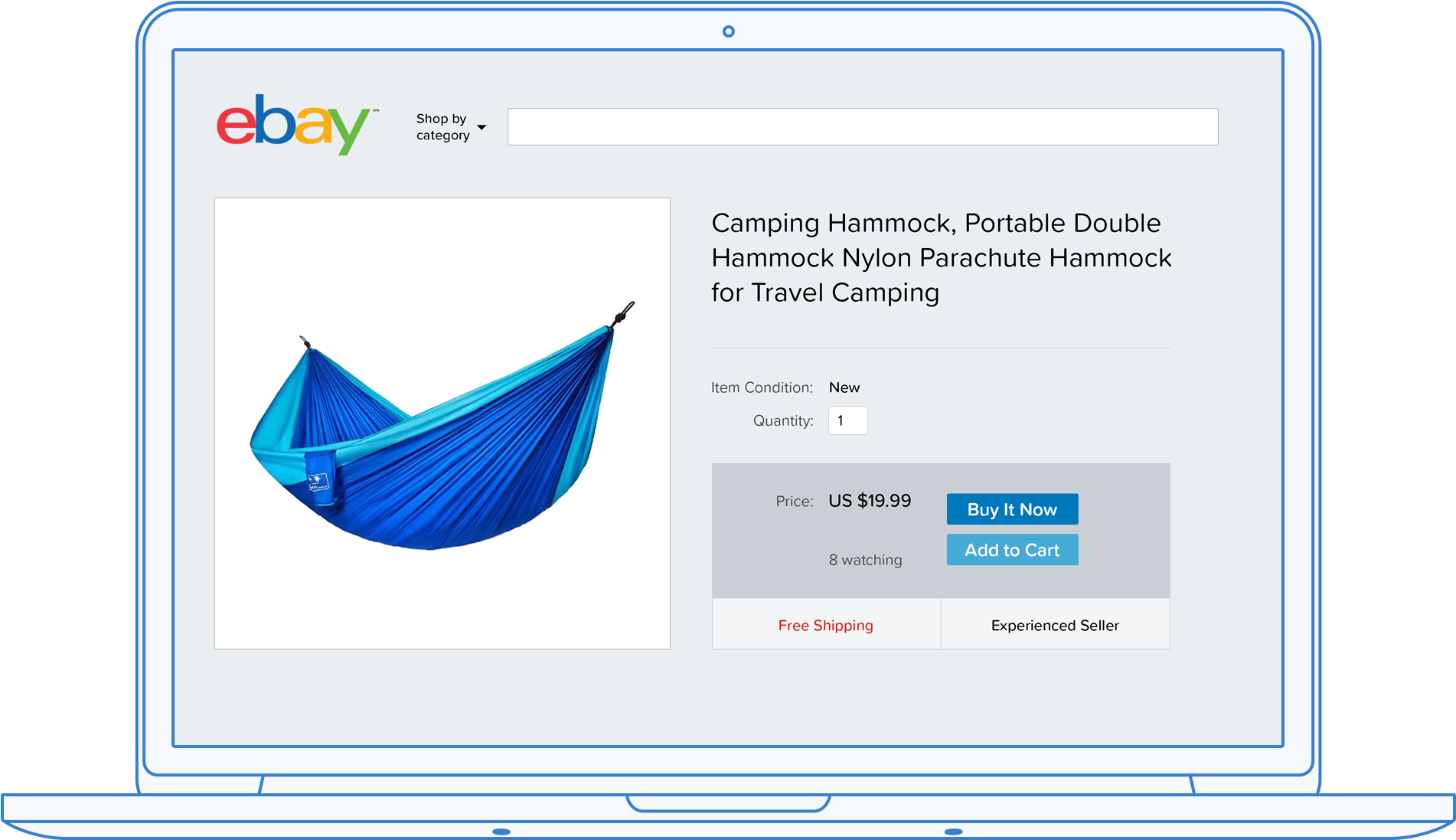This detailed and cleaned-up caption describes the nuanced features of a drawing of a laptop screen displaying an eBay listing:

---

The image features a line-drawn laptop, prominently rendered in dark blue against a grey background. The laptop is open, revealing an eBay webpage on its screen. Centrally placed at the top edge of the screen is a small dot, symbolizing the camera.

The eBay logo, in its quintessential red, blue, yellow, and green, sits in the top left corner. Adjacent to the logo on the right is a search bar. Below the eBay logo and search bar is a large, white square occupying a significant portion of this section of the screen. Inside this square is a photograph of a hammock, depicted in shades of light and dark blue, with no background context.

To the right of the hammock image, the product title reads: "Camping Hammock, Portable Double Hammock, Nylon Parachute Hammock for Travel Camping." Beneath this heading, a narrow grey line separates the title from additional text details. Although some words are unclear, it indicates that the item is "new" and lists the condition and quantity as one.

Below these details is a dark grey block displaying the price at $19.99 in US dollars. Eight users are noted to be watching this listing. The purchase options below the price include a dark blue "Buy It Now" button and a light blue "Add to Cart" button. Further descriptions below these buttons mention "Free Shipping" in red and note the seller as "Experienced" in black text on the right side.